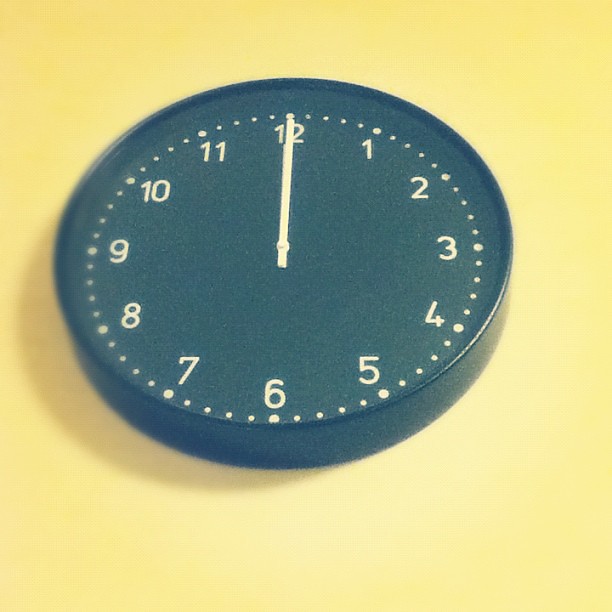The photograph captures a square image of a clock mounted on a vibrant yellow wall, which fades from darker shades at the top to lighter hues towards the bottom. The central focus is a round clock with a black plastic frame and a glossy, semi-reflective face cover, possibly made of plastic or glass. The clock face is entirely black, adorned with large, white numerals and a series of dots indicating the time, with larger dots positioned above the numbers and smaller dots in between. Both the hour and minute hands, colored white, are aligned at the 12 o'clock position, signifying either midnight or noon. The image reveals no visible second hand, possibly due to the photograph's angle or focus. The uncomplicated design of the clockface, devoid of any brand name, and the crisp alignment of the hands captured in the slight angled view, offer a minimalist yet detailed representation against the lively yellow backdrop.